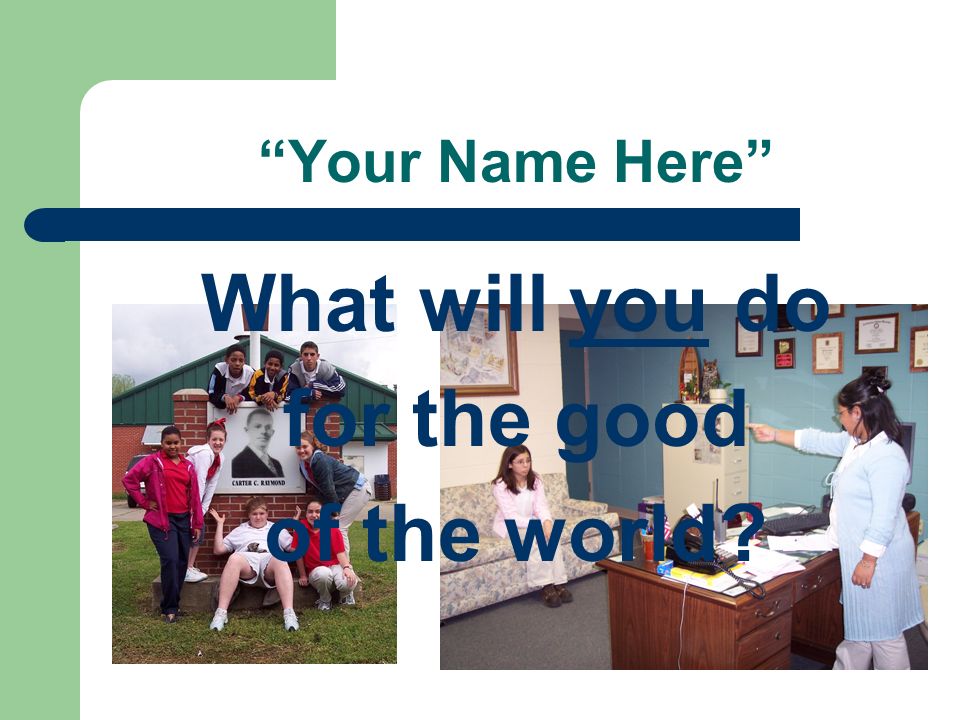**PowerPoint Slide Overview:**

The slide features a predominantly white background with a distinctive teal border running down the entire left side and extending about a third of the way across the top. This border creates a boxed-in effect at the top left corner. Positioned near the top, centered in dark green, bold text reads, "YOUR NAME HERE," each word capitalized and placed within quotation marks. Below this header, a dark blue line stretches horizontally, nearly spanning the width of the slide, stopping just short of the left and right margins (around 3% from each edge).

Just beneath this line, large, bold, dark blue text asks, "What WILL YOU DO FOR THE GOOD OF THE WORLD?" with "YOU" underlined for emphasis. This question overlays two distinct photographs side by side.

- **Left Photograph:** The image displays a group of eight children gathered around a small brick monument situated in a large grassy field, beneath a partly cloudy sky. Behind them can be seen a teal-colored house. Central to the monument is a black-and-white photograph of a man, with the name "Carter C. Raymond" displayed beneath it.
  
- **Right Photograph:** Set in what appears to be a medical waiting room, a girl in a long sweater stands behind a cluttered wooden desk, pointing towards another girl who is sitting on a sofa. The seated girl looks down at the floor, which is covered in grey carpeting. The background features blue walls adorned with various certificates. Both girls are wearing glasses, with the standing girl dressed in what resembles a nurse's uniform.

This thoughtfully arranged slide encourages viewers to reflect on their contributions to the greater good, using the evocative imagery and clear, bold text to provoke thought and inspire action.